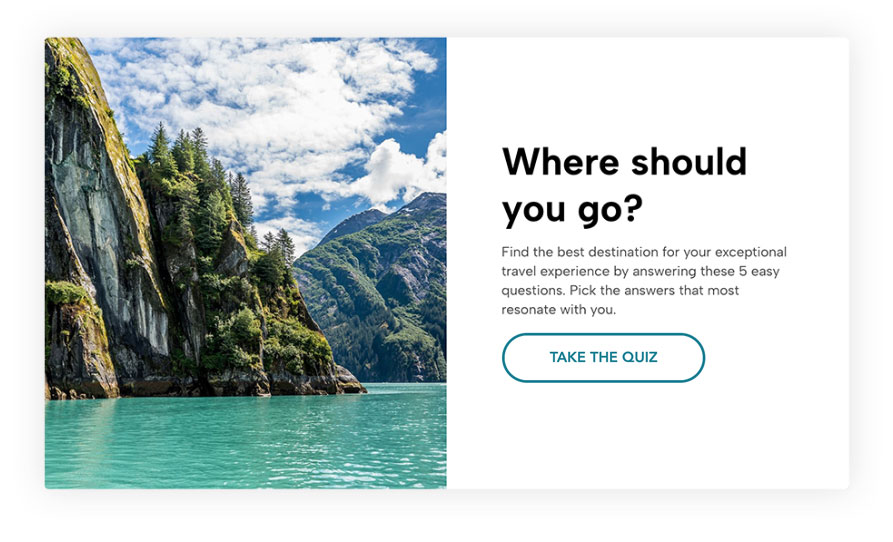The image depicts a pop-up advertisement typically found on travel websites. The left half features a stunning photograph of a body of water encircled by towering, rocky mountains under a bright, sunny sky with a few scattered clouds. The water boasts a striking bluish-green hue, adding to the scenic beauty. On the right side of the ad, against a plain white background with black text, a message reads: "Where should you go? Find the best destination for your exceptional travel experience by answering these five easy questions. Pick the answers that most resonate with you." Beneath this message, there's a noticeable "Take the Quiz" button. Overall, this is one of those disruptive pop-ups that many users often find bothersome while browsing travel websites.